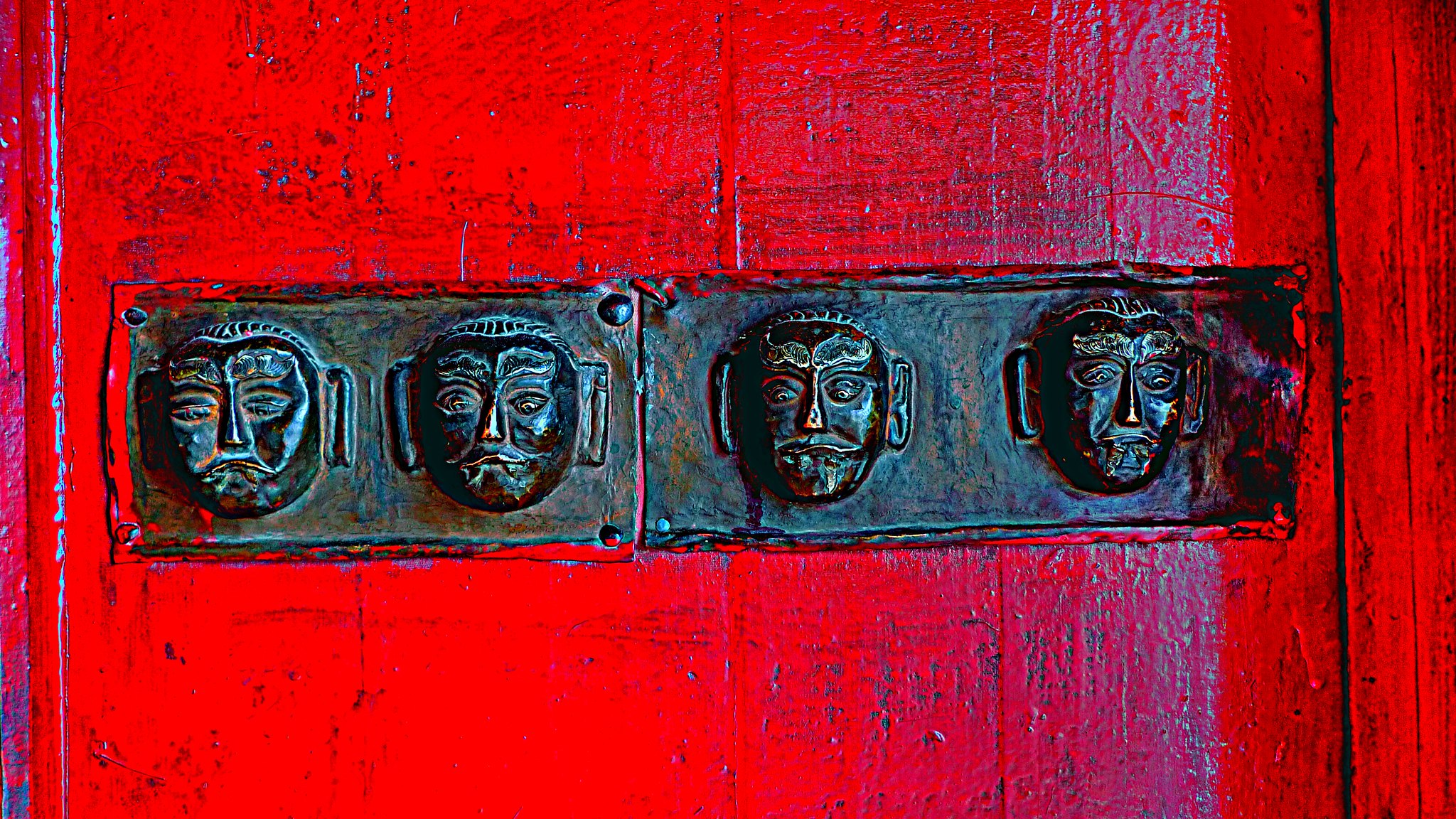The image is a vivid color photograph featuring a predominantly bright red background with wood grain texture, likely painted with glossy red paint. In the center of the image, positioned in a horizontal rectangular frame, are two metal strips or placards. These strips bear detailed engravings of four human faces, each with prominent features including well-defined eyes, noses, mouths, and eyebrows. The faces also have distinctive, large ears and some appear to be adorned with headbands, evoking an ancient cultural aesthetic, possibly reminiscent of Aztec or Mayan art. The metal faces are dark-toned and protrude outward, giving a three-dimensional effect against the ornate, glowing red backdrop with subtle hints of blue. The expressions on the faces are serious, with none of them smiling.